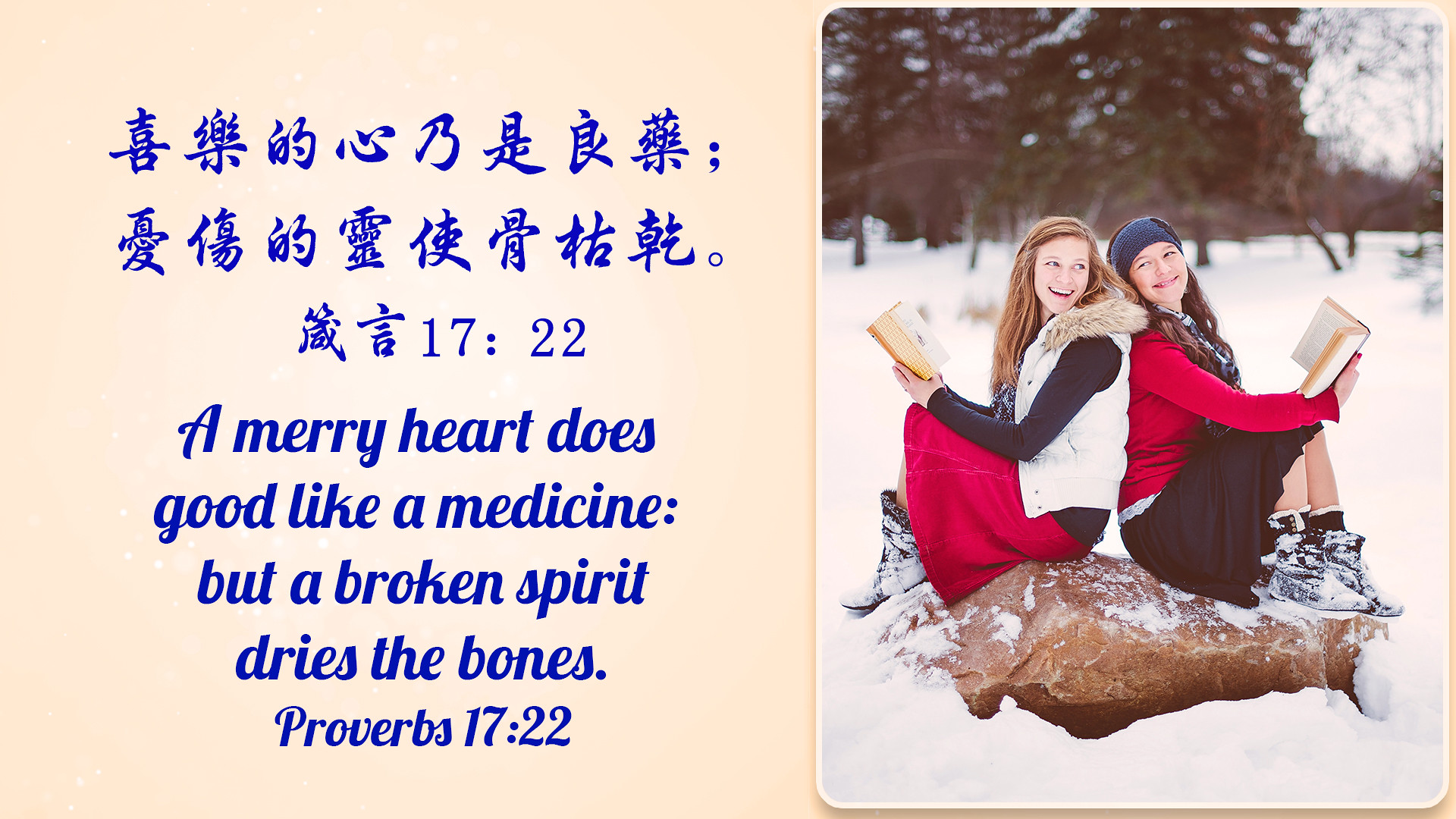In this postcard image, two young women are seated back to back on a stone in a snowy outdoor setting, each holding a book and smiling joyfully. The girl on the left, with red hair, is dressed in a white coat with a furry collar, a red skirt, and a black shirt. Her counterpart on the right wears a red shirt, a black skirt, and a blue bandana over her hair. Both girls have snow covering their boots, and distant trees add depth to the winter scene. The right-hand side of the postcard is occupied by this vivid photo, while the left side features two and a half rows of Chinese characters followed by a paragraph of blue English text against a beige background. This text reads, "A merry heart does good like a medicine, but a broken spirit dries the bones. Proverbs 17:22." The overall design of the postcard, with its blend of imagery and motivational message, evokes a festive and heartwarming atmosphere.